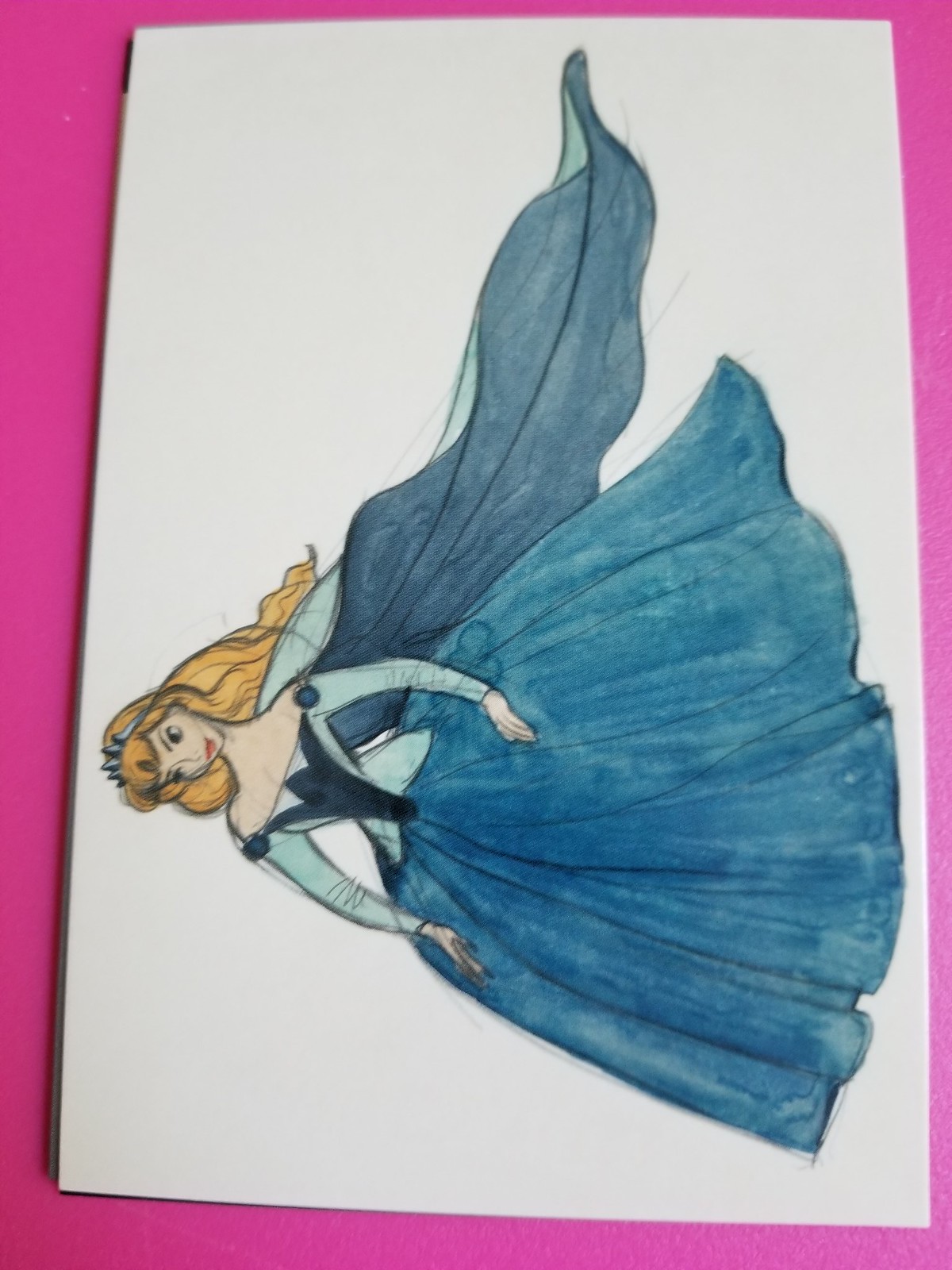The photograph features a detailed colored pencil drawing on a thick piece of paper, oriented sideways on a vibrant hot pink or pinkish-purple surface. The sketch portrays a Disney-like princess, strikingly reminiscent of Aurora from "Sleeping Beauty," highlighted by her facial features, long flowing blonde hair, and regal attire. She is adorned with a tiara and makeup, exuding a happy demeanor with her head slightly tilted. Her elaborate gown features a dark blue bodice, light blue sleeves, and intricate dark blue lines and circles on the lighter blue areas, evocative of a 1950s style. The dress flares out at the bottom, transitioning into a voluminous dark blue skirt with distinctive lines. Complementing her ensemble is a majestic cape flowing from her shoulders, light blue on top and dark blue beneath, accentuated by black lines.